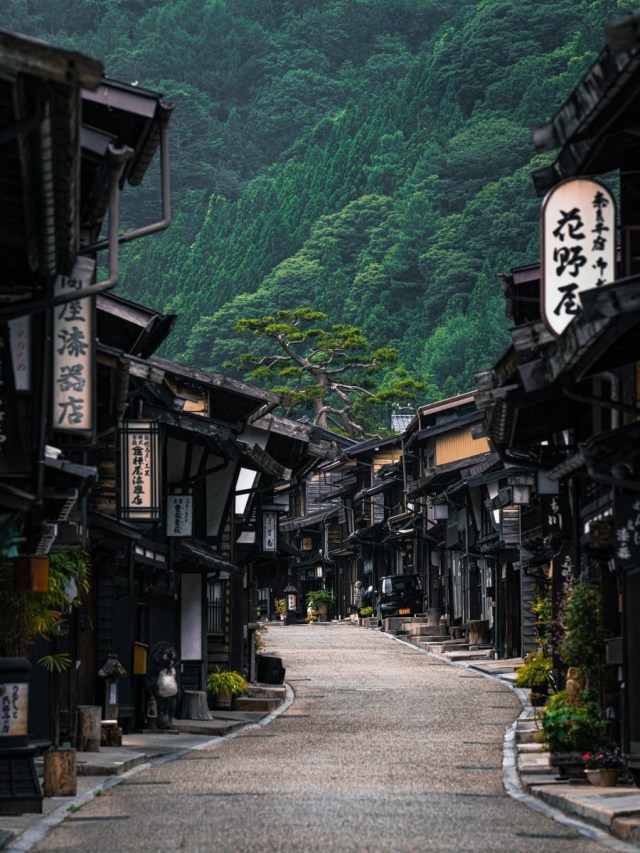This vertical rectangular image depicts a narrow, winding street in an ancient Asian town, possibly in a mountainous region of Japan. The path, which appears to be made of stone or gravel, meanders through closely packed, dark wooden buildings that evoke a traditional, old-world aesthetic. Numerous structures feature white banners with black Oriental characters, suggesting they could be storefronts or homes. The street is devoid of vehicles and emphasizes pedestrian movement. On the right side of the image, one building has a collection of potted plants outside. The buildings are dark and quaint, reminiscent of Swiss chalets. Above them, a finely trimmed bonsai-like tree adds artistic contrast to the scene. Dominating the background, a towering, green mountainside covered in dense foliage fills the upper part of the photograph, creating a dramatic natural backdrop.